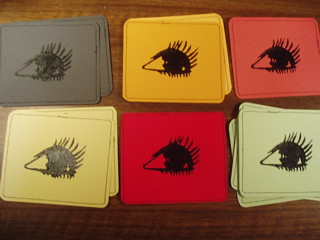The photograph captures an aerial view of several colorful cards laid out on a dark brown wooden table. The cards are organized into six somewhat haphazard piles. 

- The top left pile contains at least two cards, primarily grey in color.
- The top center pile has two cards, both in a yellowish-orange hue.
- The top right pile consists of a single pink card.
- The lower left pile includes at least two yellowish cards.
- The lower center pile has a single red card.
- The lower right pile features at least three, possibly more, mint green cards.

Each card has a thin black border and displays an illustration of a small, furry creature. The creature has a triangular, bare head and a round, hair-covered body, somewhat resembling a hedgehog.